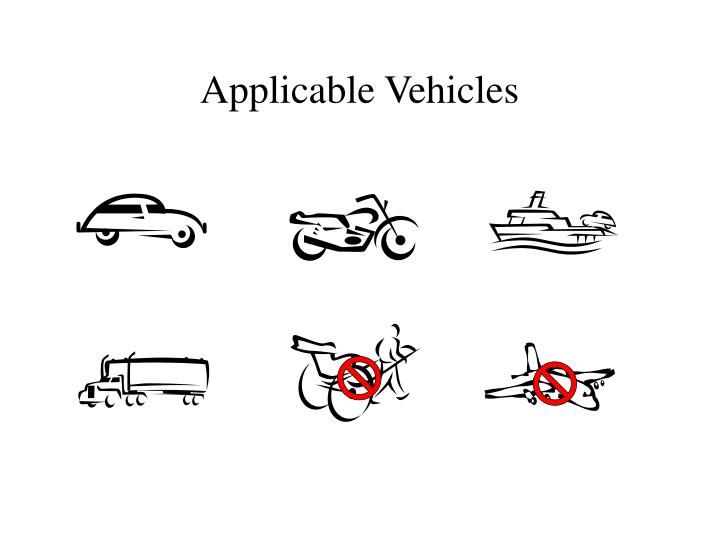The image displays a white background with the title "Applicable Vehicles" at the top in black text, with both 'A' and 'V' capitalized. Centered on the image are six line-drawn, uncolored sketches of various modes of transportation, arranged in two rows of three. The top row features a side view of a car facing right on the left, a motorcycle in the middle, and a boat on the right. The bottom row includes a semi-truck facing left on the left, a person pulling a two-wheeled cart or rickshaw in the middle with a red circle and slash indicating it is not allowed, and an airplane on the right also marked with a red circle and slash indicating it is not allowed.